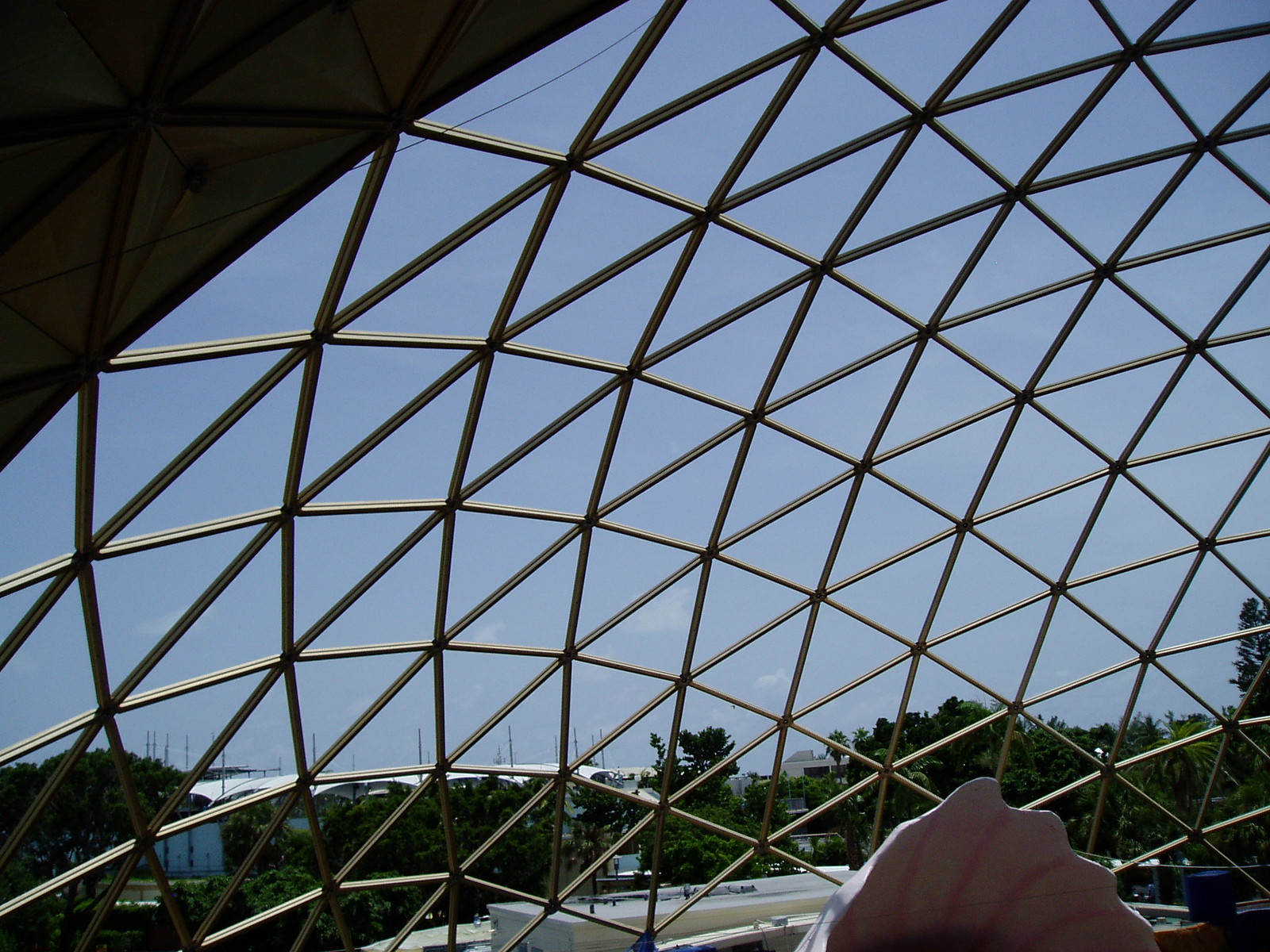The photograph depicts an outdoor scene taken from behind an intricately designed, domed observation deck featuring a clear, protective mesh in a triangular pattern. The oval structure creates a partially open roof through which the sky is visible. In the distance, a vast expanse of trees is noticeable, along with various urban elements like telephone poles, street lights, and rooftops of some flat homes. The sky is light blue with a few small clouds. Positioned in the bottom right corner of the image is a large, shell-like object with a pinkish hue, giving the impression of being in an amusement park or perhaps a uniquely designed public space. The overall atmosphere conveys a blend of natural scenery and urban landscape, viewed from a height that makes the viewer feel as though they could almost touch the wire mesh.